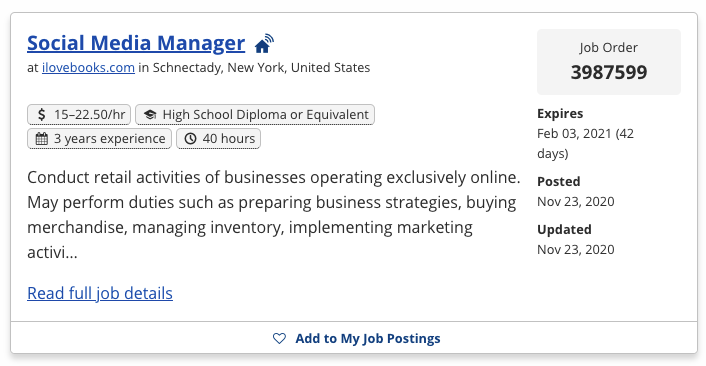The image is a detailed job posting for a Social Media Manager prominently displayed at the top in blue text. Adjacent to the title, there's an icon of a house with a Wi-Fi symbol above it, indicating that the job is remote. Below the title, it specifies the website "ilovebooks.com" and mentions that the company is based in New York, United States.

Further down, various icons present job requirements and details. One icon shows a dollar sign with the pay rate listed as $15 to $22.50 per hour. Next, there's a graduation cap symbol denoting that a high school diploma or its equivalent is required. Following that, a calendar icon specifies that candidates should have three years of experience. Another icon illustrates a clock, indicating a full-time commitment of 40 hours per week.

The textual part of the posting describes the job's responsibilities, including conducting retail activities for businesses that operate exclusively online. Responsibilities also entail preparing business strategies, purchasing merchandise, managing inventory, and implementing marketing activities, among others, with the description cut off by an ellipsis. A blue link at the end invites users to "Read full job details."

On the right side of the image is the job order number, 3987599, displayed in a gray box with black text. Below this, it notes that the job expires on February 3rd, 2021, which was 42 days from the posting date of November 23rd, 2020—the same date it was updated. At the very bottom of the image, there's a heart icon and the option to "Add to my job postings."